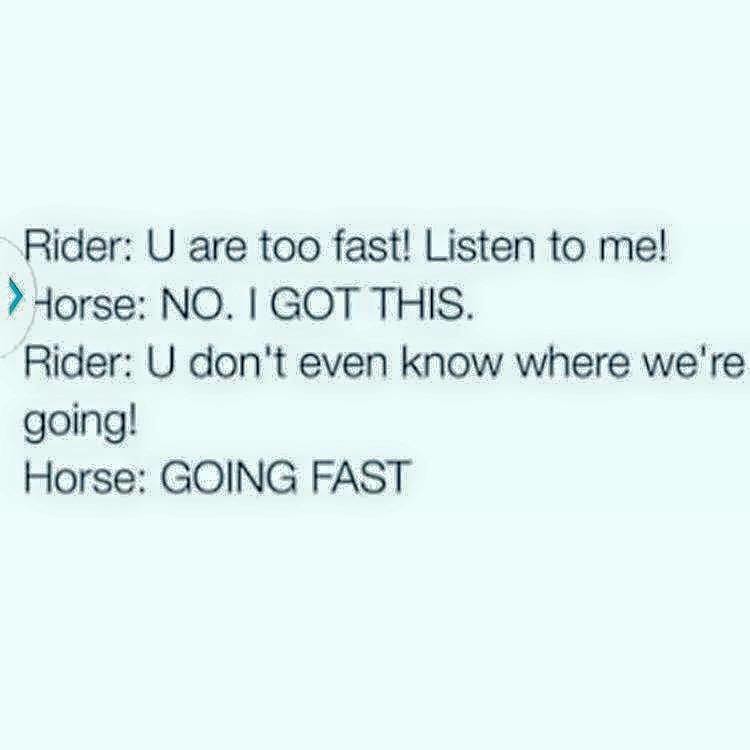The image features a light blue background with a semi-circle and a right-pointing arrow symbol in the upper left corner, suggesting it might be from a user interface on a phone or computer. The text, presented in black sans-serif font, mimics a fictional conversation between a rider and a horse. The dialogue reads:

"RIDER: You are too fast! Listen to me!
HORSE: NO! I got this.
RIDER: You don't even know where we're going!
HORSE: GOING FAST."

The horse's responses are highlighted in all capital letters, adding emphasis and humor to the exchange by portraying a spirited and determined horse rebelling against its rider's attempts at control.